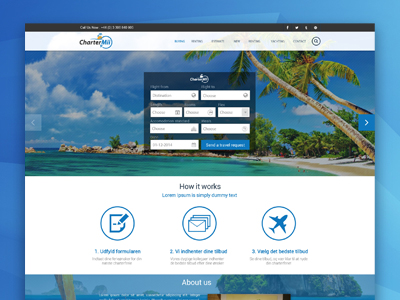This image is a screenshot of a web page for Charter MN, a travel agency. In the screenshot, the Charter MN window is not in full-screen mode, allowing the computer's desktop background to be visible behind it. The desktop background consists of geometric shapes in varying shades of blue.

The Charter MN web page features a sleek black ribbon at the top, followed by a thicker white ribbon displaying the program name. Below this is the main section of the web page, which offers various options for booking travel. The page's background image showcases a picturesque beach scene with palm trees, the ocean, and the shore stretching into the distance.

Superimposed on this background image are fields for inputting trip details. Beneath this section is another white ribbon bar, occupying about a quarter of the total screen area, which outlines the process of booking a trip with Charter MN. It illustrates steps such as booking the trip, receiving a confirmation email, and eventually traveling.

Further down the page is the "About Us" section, offering more insight into the services and mission of Charter MN.